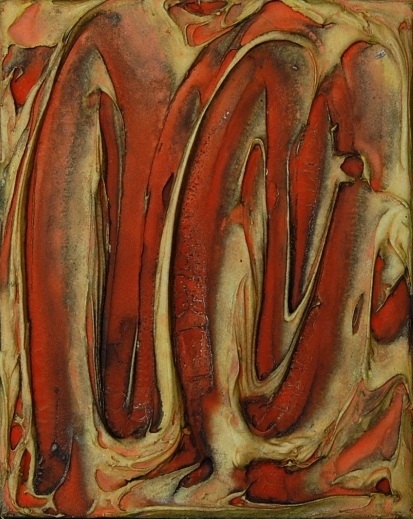This intriguing abstract oil painting on a tall rectangular canvas features a mesmerizing interplay of curving oval shapes and dynamic brushstrokes. Dominated by various shades of red, pink, yellow, and brown, with contrasting touches of black, white, and gray, the artwork creates a complex, washed-out yet captivating visual experience. The background appears to be a tan hue, upon which heavier applications of rust-red and brown oil paints are swirled and marbled, producing thick and chunky textures. These substantial brushstrokes blend and bleed into each other to form lighter shades and intricate patterns, reminiscent of intestines or coiled snakes, evoking the impression of muscles and tendons. Despite its abstract nature, some viewers might perceive faint suggestions of letters or human forms within the curves. The lack of a signature, title, or any text further invites the viewer into a purely imaginative interpretation of this truly enigmatic piece of art.